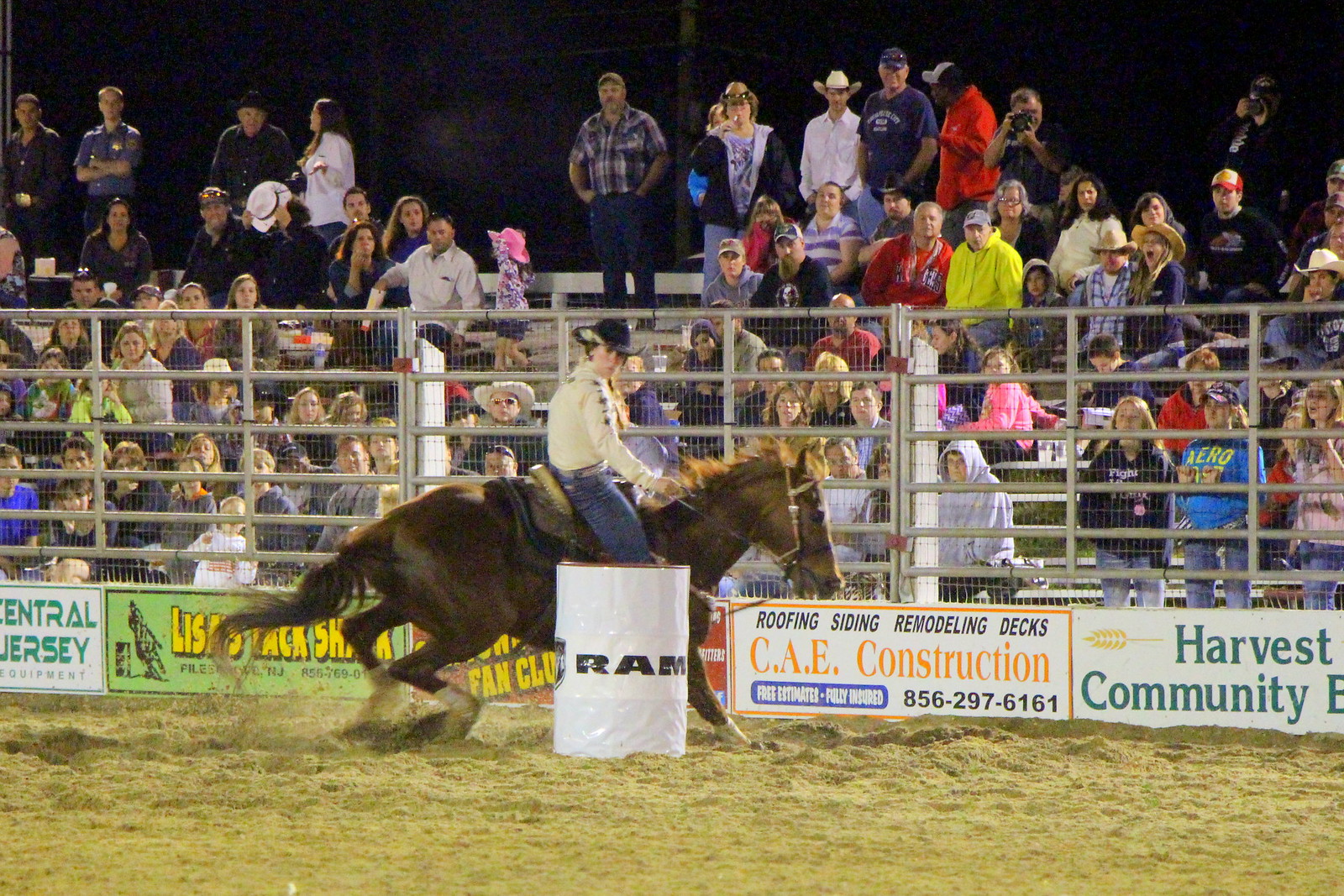This nighttime rodeo photograph captures a young woman riding a brown horse in the midst of a barrel race. She is dressed in a brown button-down shirt, blue jeans, and a black cowboy hat. The brown horse, equipped with a saddle, is navigating around a white barrel emblazoned with the word "RAM." The ground is covered with loose, sawdust-like dirt. Surrounding the arena, a silver metal fence barrier topped with advertisements stands between the dirt track and a full stadium of spectators. One prominent advertisement at the bottom reads "Harvest Community," while another visible one denotes "Roofing, Siding, Remodeling, Decks, CAE Construction," with a phone number "856-297-6161." The audience, extending up several stories, is a large crowd of spectators, mostly seated, with some standing. Against the backdrop of a completely black night sky, the scene captures the energy and preparation inherent in this competitive event.